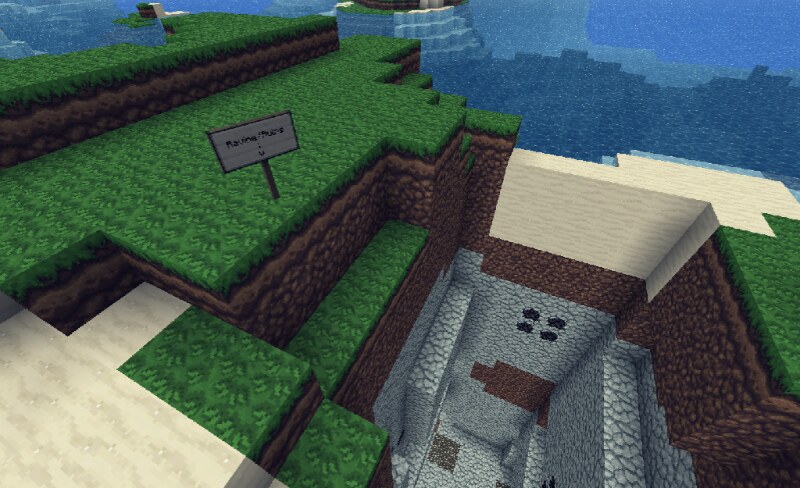The image appears to be a scene from the game Minecraft, showcasing a diverse and tiered landscape. In the background, various shades of blue suggest the presence of water, transitioning from lighter to darker blues. The terrain is composed of multiple layers, with vibrant green grass covering the topmost surface. Beneath the grass, several brown dirt layers are visible, representing the earth.

On the left side of the image, the highest terrain level gradually descends into a broader, substantial platform. This platform then drops again, creating a green-covered ledge. To the right, the landscape features a light brown, beige area that intersects with the water, resembling a sandy beach or shoreline. This sandy area seamlessly transitions into a grassy expanse further to the right.

Centrally, a significant excavation is evident, revealing a subterranean layer of solid gray rock. Scattered within this rocky layer, a few black specks indicate the presence of valuable resources or minerals, characteristic of Minecraft's mining elements. The overall scene intricately displays the game's iconic, blocky environment, highlighting different natural elements and terrain variations.